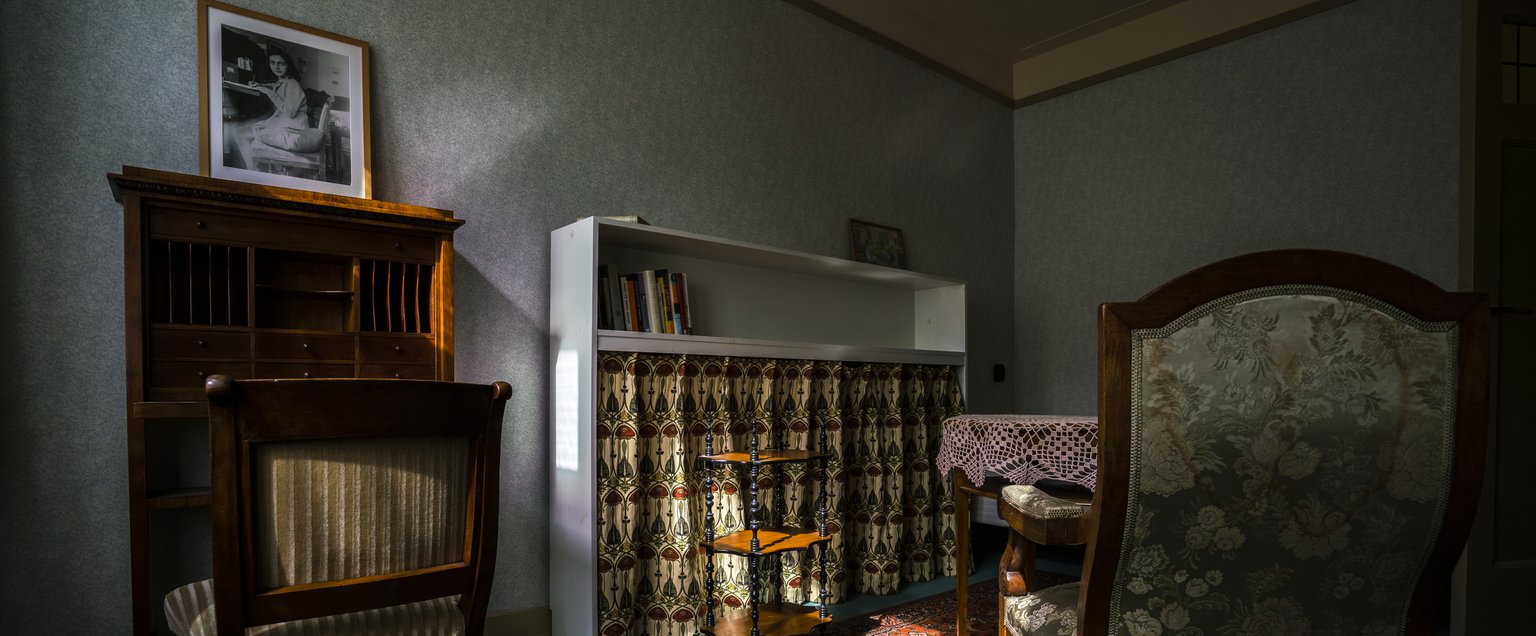This image captures a section of what appears to be an old-fashioned interior, potentially from the 1920s, focusing primarily on the corner of the room. The ambiance is reminiscent of a study or a small living space, characterized by its vintage aesthetic. There is a prominent wooden chair with green brocade and flower embroidery, suggesting an air of elegance. Nearby stands a small wooden table, adorned with a delicately patterned lace crochet doily. 

A white bookshelf occupies part of the scene, with its lower sections concealed by a curtain, while the visible shelf holds only a few items. In front of this bookshelf is a three-tiered side table. To the left, another wooden chair is pulled up to what looks like a desk. The desk and bookshelf both hold framed photographs, one of which prominently features a woman, likely Anne Frank, given the context of the Anne Frank House in Amsterdam. The walls are covered in light gray wallpaper with a cream-colored border separated by a wooden strip. The intricate details and aged furnishings evoke a bygone era, adding to the evocative memory of the space.